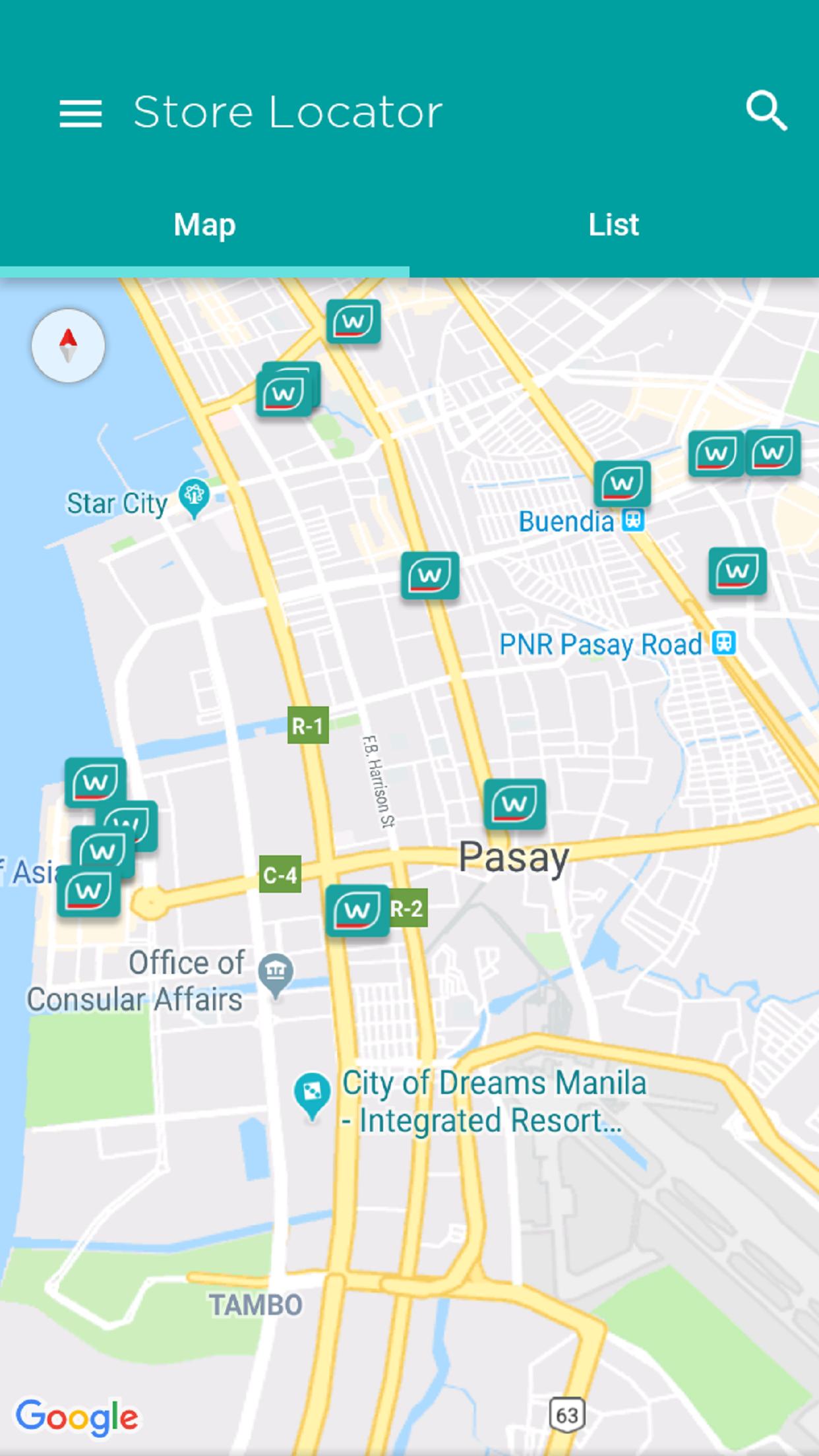Screenshot of a store locator app interface with a search function and view options

The screenshot captures the interface of a store locator app. At the top, the header displays the words "Store Locator," accompanied by a magnifying glass icon on the right, indicating a search function. Below the header, there are two tabs labeled "Map" and "List," with the "Map" tab currently selected. The map view shows a geographical area situated close to a body of water. Multiple markers are seen on the map, with one prominently highlighting the location labeled "Star City" in Pasay. The map provides an intuitive visual guide to nearby stores, enhanced by the app's navigational features.